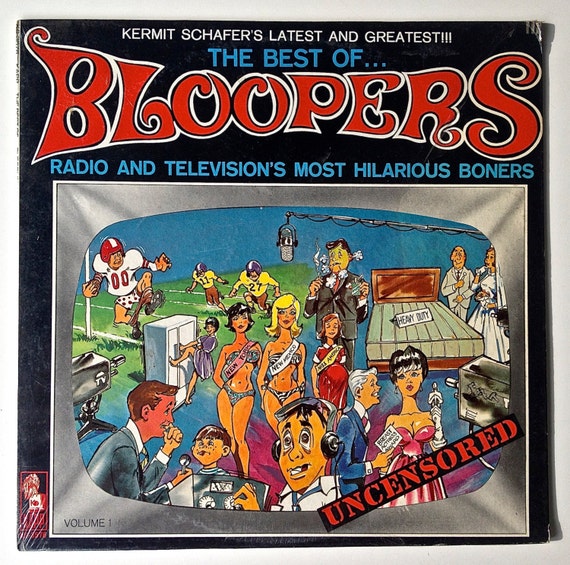This image is an advertisement, likely a page from a magazine or a record cover, featuring a black background. At the top, the text in white reads, "Kermit Schafer's latest and greatest!!!" Below it, "the best of..." is printed in blue, followed by "bloopers" in large red letters with a white border. Additionally, in blue text, it states "radio and television's most hilarious boners." The illustration below is quite busy, incorporating various humorous cartoon elements. A silver-outlined television displays a central microphone, surrounded by scenes of football players, including one with his pants down, announcers, women in bikinis, a pregnant woman in a beauty pageant sash, a host interacting with a young boy stifling laughter, and a woman struggling with a cabinet. There's also a bed labeled "heavy duty," a bride and groom, and multiple cameras capturing the chaotic scenes. At the bottom, "uncensored" is prominently displayed in red print.